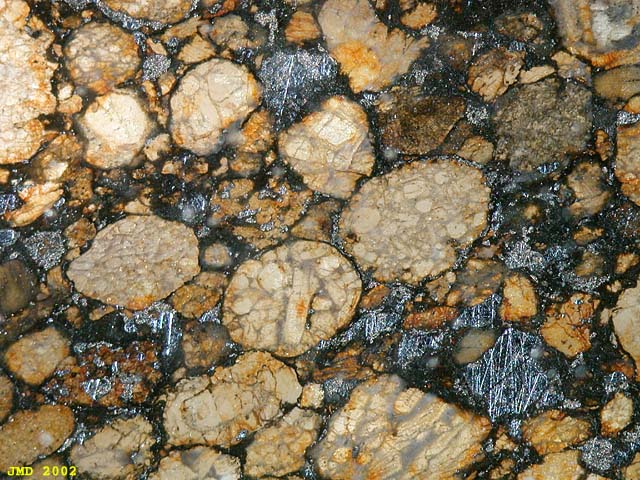The image captures an overhead view of a complex rock surface that evokes the texture and appearance of a dried-up ocean floor. Various types and colors of rocks dominate the scene, some displaying a scratchy pattern reminiscent of underwater formations. In the bottom right, several black stones feature an up-and-down scratching pattern that resembles lifelines. In contrast, the top left showcases clear, beige stones adorned with small circles and unique patterns. Interspersed throughout the surface are smaller rocks, including a striking red stone on the bottom left, which also exhibits the scratchy texture seen on the black rocks. Additionally, the bottom left corner features yellow text that reads "JMD 2002," adding a human element to this natural tableau. The entire composition, possibly captured with a digital camera during daylight in a forest or similar setting, highlights the diverse textures and colors, encapsulated in a black substance veined with white outlines.